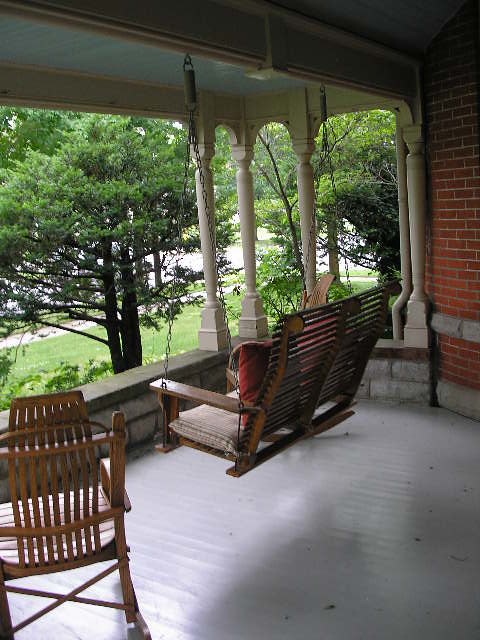This photo captures a picturesque front porch scene. The house is made of red brick with a white-painted wooden porch floor extending outward. The porch is supported by slender white columns that reach up to the roof, which creates a shaded, cozy nook. A wooden swinging bench, suspended by chains from the roof, features a vibrant red pillow, adding a pop of color. Next to the swing, there is a classic wooden rocking chair. The view beyond the porch showcases a lush front yard with vibrant green grass and various shades of green in the tall, leafy trees. A concrete walk path cuts through the greenery. The image is taken during the daytime, where the bright outdoor light contrasts with the cool, shaded area under the porch roof.